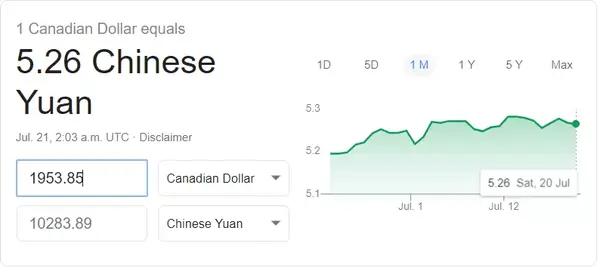The image provides a detailed conversion of Canadian dollars (CAD) to Chinese Yuan (CNY) against a minimalist white background. At the top, in light gray text, it states "1 Canadian Dollar equals," followed by a prominent black text showing "5.26 Chinese Yuan." Beneath this, a smaller, light gray caption reads "July 21st, 2:03 a.m. UTC, disclaimer." Below these details, two conversion boxes are displayed: one indicates 1,953.85 CAD, which converts to 10,283.89 CNY.

Adjacent to these boxes on the right, there is an informative graph illustrating the exchange rate trends. The horizontal axis at the top of the graph is labeled with time options: "1 day," "5 days," "1 month," "1 year," "5 years," and "Max." The bottom of the graph features a timeline starting from "July 1st" to "July 12th," and the data points extend up to "Saturday, July 20th." The visual representation assists in understanding the historical exchange rate movements over various periods.